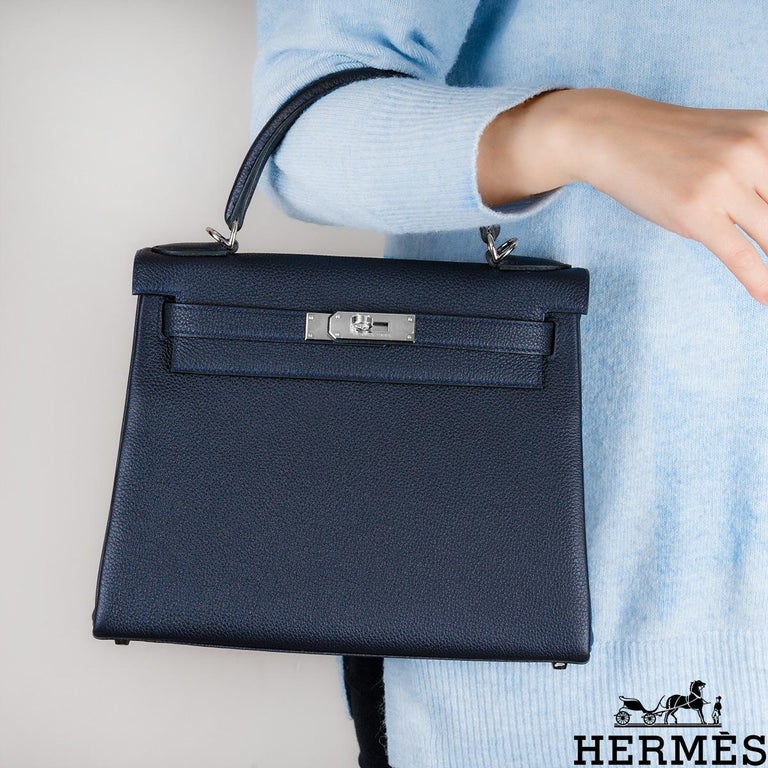This advertisement photo for Hermes features a close-up shot of a sophisticated, black trapezoid-shaped handbag made from dimpled, textured leather. The purse boasts a stiff, semi-circle handle with brass connections and a metallic silver clasp positioned at the center top. The bag's understated elegance is complemented by its simplicity and mid-sized design, ideal for everyday use. The handbag is draped over the arm of a woman, who is wearing a very light blue, Carolina blue, simple long sweater. Only the upper portion of her hand and wrist are visible, with her arm bent at a 90-degree angle. The composition focuses on the luxurious purse and the lower part of her arm, creating a sense of refined style. At the bottom right corner of the image, the iconic Hermes logo is prominently displayed, featuring a black silhouette of a horse pulling a carriage, with a man in riding gear standing in front of it.